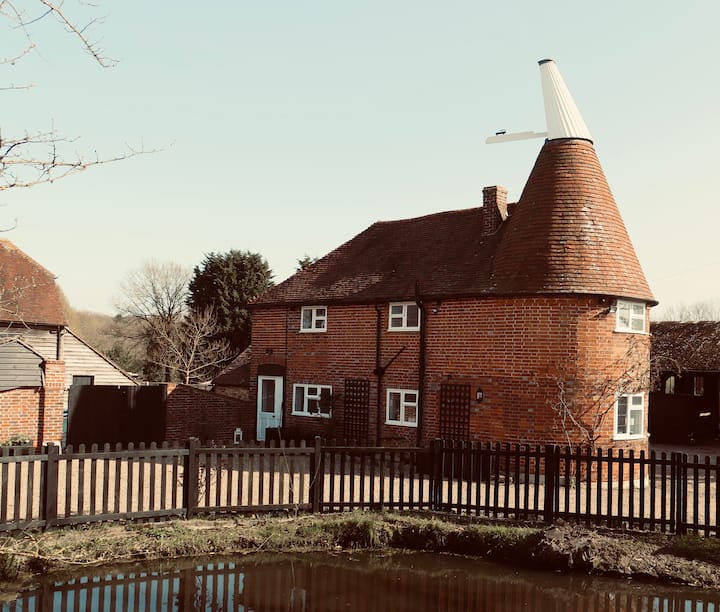In this outdoor photograph, a fenced, small muddy pond occupies the bottom portion of the image, surrounded by overgrown grass and weeds. The brown wooden fence encloses the pond, beyond which is a dirt walkway. There is a brick house to the far left outside the fence, and the main focus in the center is a red brick building with a distinctive architecture. This building features a combination of a cone-shaped roof and a larger, pyramid-shaped section, both topped with brown roofing. The brick structure includes numerous white-framed windows and a white door, adding to its striking appearance. Further to the right, another house is barely visible down the pathway. In the background, trees border the scene, some bare and others retaining their green foliage. The sky transitions from a milky white near the horizon to a clearer blue above, suggesting that the photo was likely taken in the early morning.